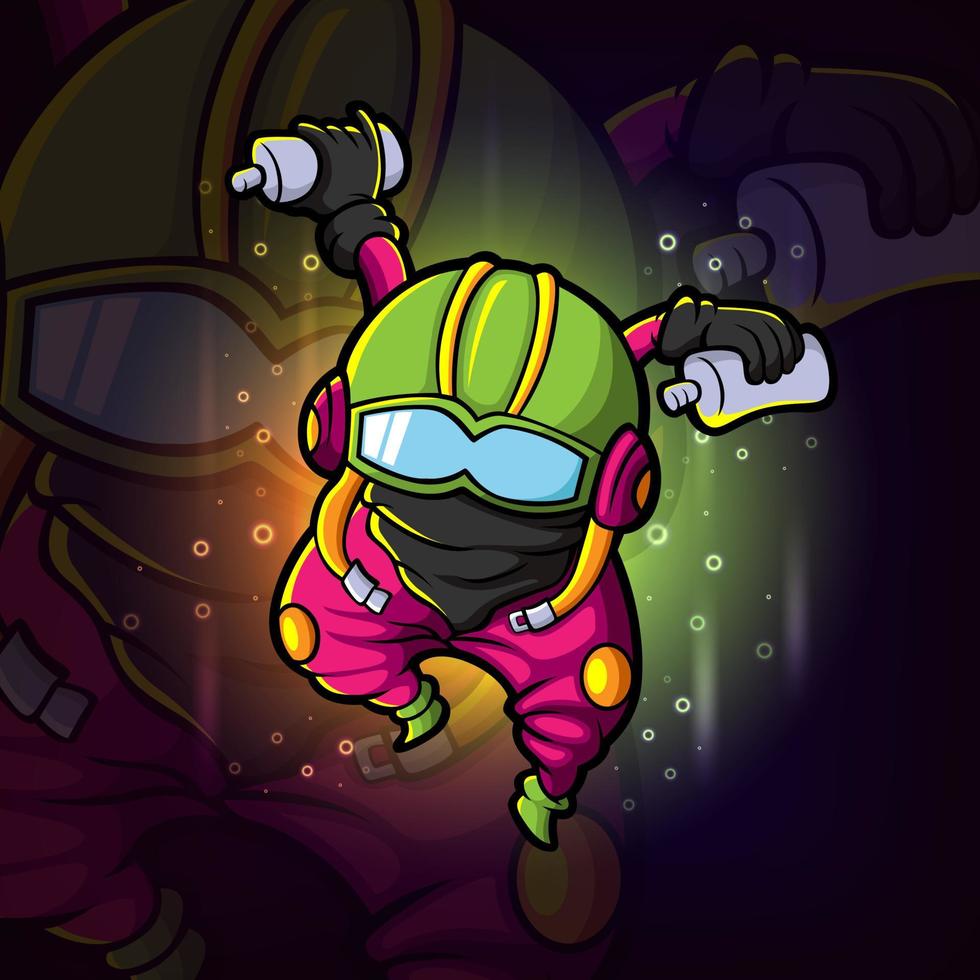This is a cartoon drawing of a peculiar, futuristic character that resembles a squished person or a small alien. The character appears to be jumping or swimming forward. It has a distinctive helmet that's primarily green with a design reminiscent of a fighter jet pilot's helmet, featuring blue ski goggles outlined in green and two disconnected central pipes resembling rib bones. At the sides of the helmet are circular, purple ear cups, each with an orange seatbelt strap dangling from it.

The character's body below the helmet is clad in a black turtleneck-like garment that covers its entire neck and face. Its arms, which are the same pink-purple color as its pants, are raised above its head and each hand, covered in black gloves, holds a bottle similar to a shampoo or spray paint bottle.

The character’s lower half is dressed in pink, baggy pants with some orange and yellow circular patches on the knees, giving the impression of genie pants. It has tiny green feet that resemble socks covering small, triangular feet with no visible toes.

A faded, larger version of the same character is superimposed in the background, creating a layered visual effect. Surrounding the character are faint circles and lines, resembling bubbles or Cheerios, contributing to an underwater or ethereal atmosphere. 

The vivid colors and detailed elements highlight the artistic nature of the piece, suggesting a creation of a fictitious, possibly alien, futuristic character.